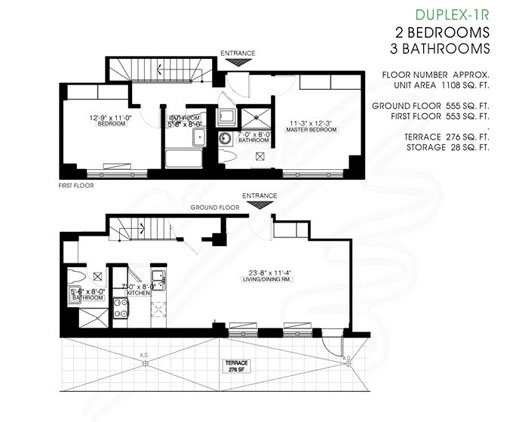This image is a detailed floor plan for Duplex 1R, featuring a combination of two and three-bedroom configurations. 

At the top right corner, the label "Duplex 1R" is highlighted in green. The floor plan specifies a total approximate unit area of 1,106 square feet, divided into a ground floor of 555 square feet and a first floor of 553 square feet. Additionally, the plan includes a terrace area measuring 276 square feet and a storage space of 28 square feet.

The layout begins at the first floor, where the entry point is marked by an arrow pointing downwards. On the left-hand side, the first bedroom measures 12 feet 9 inches by 11 feet 0 inches. Adjacent to this bedroom is the bathroom. Continuing to the right, the master bedroom spans 11 feet 3 inches by 12 feet 8 inches and includes a small en-suite bathroom measuring 7 feet 8 inches by 8 feet 8 inches.

Moving down to the ground floor, the layout features a generous living area on the right side, which measures 12 feet 8 inches by 11 feet 4 inches. On the left side of the ground floor, there is a kitchen adjacent to another bathroom. The front portion of the ground floor provides access to a spacious terrace area.

Overall, this meticulously detailed floor plan offers a comprehensive view of the duplex unit, highlighting each room's dimensions and the functional layout of both floors.